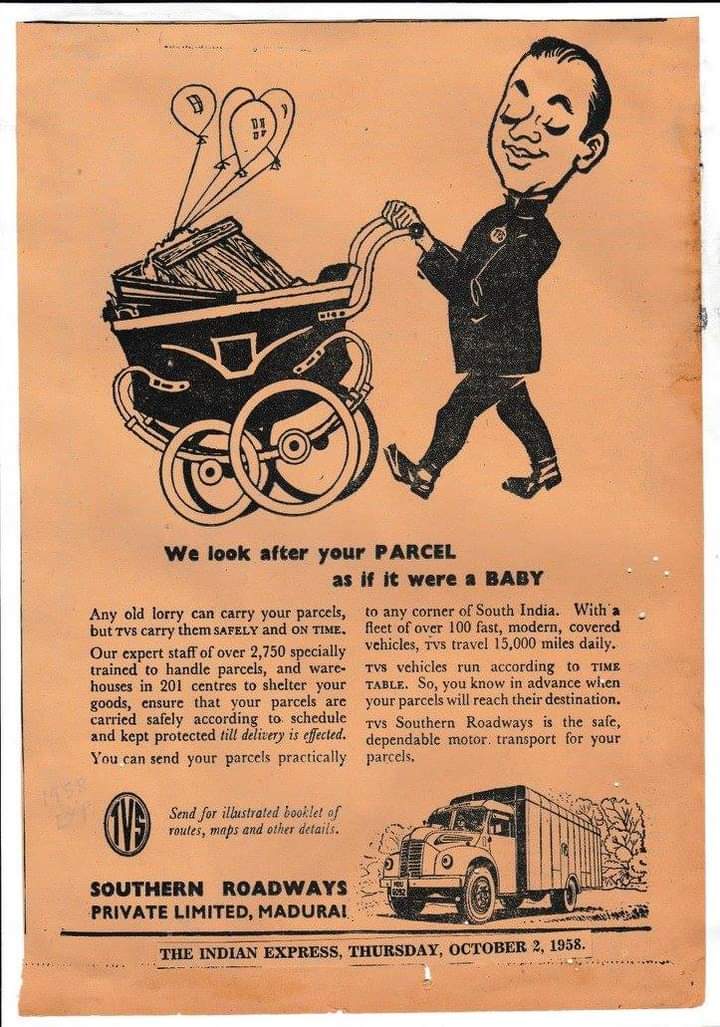In this vintage advertisement from "The Indian Express" dated Thursday, October 2nd, 1958, the paper is a distinct orange color, which may have either been its original hue or a result of aging over time. Dominating the top of the image is an intricate black-and-white drawing depicting a man in a bellboy uniform pushing a cart filled with balloons. The man faces left, his eyes closed in a gentle smile. Below this illustration, a prominent slogan reads, "We look after your parcel as if it were a baby."

The advertisement further elaborates on the exceptional services provided, stating, "Any old lorry can carry your parcels, but TVS carries them safely and on time." It highlights the expertise of over 2,750 specially trained staff members, alongside numerous warehouses designed to shelter goods, ensuring the utmost safety and punctuality for parcel deliveries. Additional text invites readers to send for a booklet detailing routes, maps, and other information from Southern Roadways Private Limited, located in Madurai.

At the bottom of the image, on the left, the company name "Southern Roadways Private Limited, Madurai" is clearly indicated, while a small drawing of a truck appears on the bottom right. Finally, the newspaper's title "The Indian Express" and the date, "Thursday, October 2nd, 1958," are neatly positioned at the bottom, framing this nostalgic and detailed advertisement.